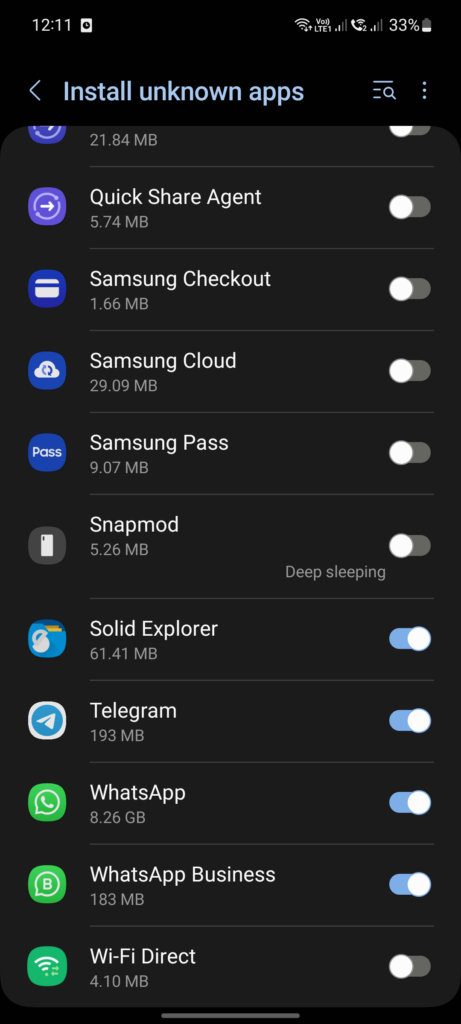This image is a detailed screenshot from a person's cell phone with a black background. The time displayed at the top left corner is 12:11. To the top right, a battery icon shows 33% remaining battery life. Beneath these indicators is the title "Install Unknown Apps".

The screenshot features a list of apps, each with its respective memory usage in megabytes (MB), with some radio buttons selected, indicating apps where installation from unknown sources is enabled. The apps listed are as follows:

1. **Quick Share Agent - 5.74 MB**
2. **Samsung Checkout - 1.66 MB**
3. **Samsung Cloud - 29.09 MB**
4. **Samsung Pass - 9.07 MB**
5. **SnapMod - 5.26 MB**
6. **Deep Sleeping**
7. **Solid Explorer - 6.41 MB** (Radio button selected)
8. **Telegram - 193 MB** (Radio button selected)
9. **WhatsApp - 8.26 GB** (Radio button selected)
10. **WhatsApp Business - 183 MB** (Radio button selected)
11. **Wi-Fi Direct - 4.10 MB**

The image is significantly taller than it is wide and does not include any human figures.